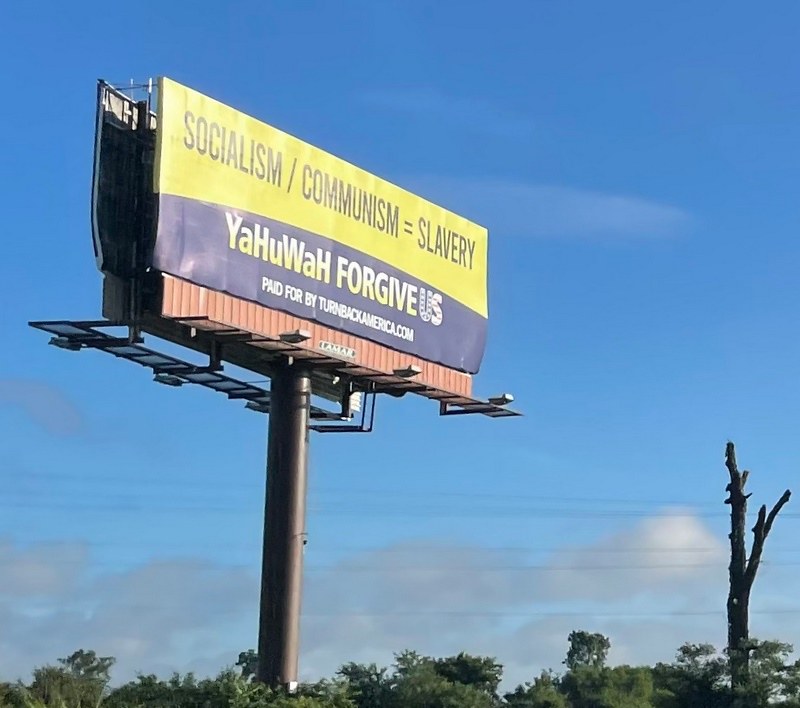The photograph captures a striking scene likely taken from an interstate or highway, though the road itself is not visible. Dominating the image is a large billboard positioned slightly to the left of the center. The billboard is elevated on a black steel cylindrical pole, leading up to the expansive advertisement surface.

The top portion of the billboard is a vivid yellow with blue lettering, bearing the provocative message: "Socialism / Communism = Slavery." Below this, a dividing line separates the upper section from the bottom section, which features a blue background with yellow lettering stating: "WAYAHUWAH forgives forgive us." At the very bottom, there is some small text that reads, "Paid for by [indistinct] southern.com," though the exact wording is difficult to decipher.

The backdrop of the billboard scene is a picturesque blue sky dotted with a few clouds. In the bottom right corner of the photograph stands a stark, leafless tree, appearing almost black. Additionally, a line of green trees stretches across the bottom of the image, adding a touch of nature to the otherwise industrial scene.